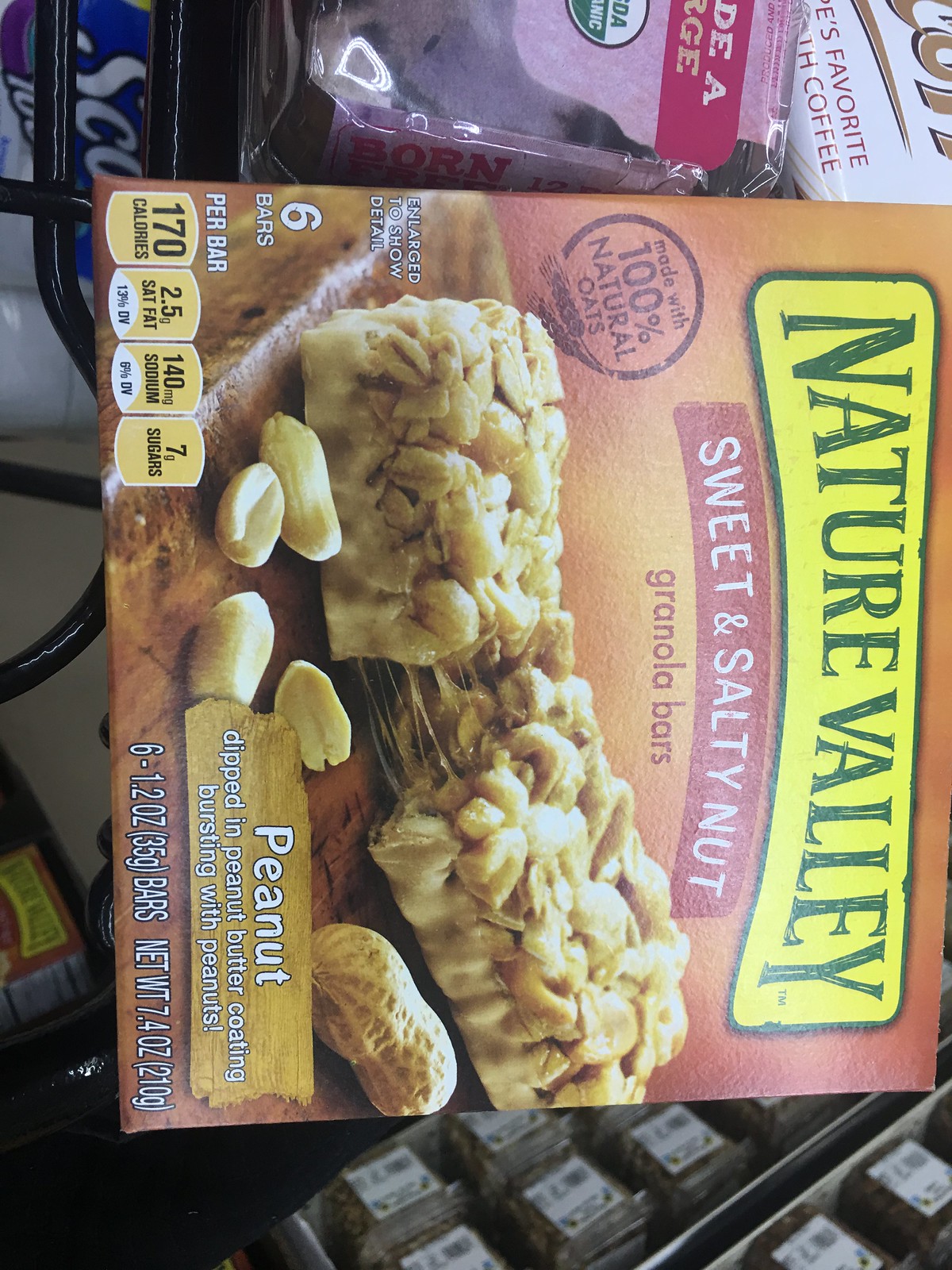This close-up color photograph showcases a rotated package of Nature Valley Sweet and Salty Nut Granola Bars. The box, prominently beige-brown with accents of orange, features the brand's iconic yellow curved rectangle logo with "Nature Valley" written in dark green. Below it, a red banner with white text reads "Sweet and Salty Nut." The image of the granola bar, visibly tan with whole peanuts and a gooey filling being pulled apart, dominates the center. Nutritional information and weight details appear at the bottom right corner in white text. Surrounding the main package, the background contains various indistinct food items, including a white and gold package and a pink and clear plastic package in the upper right corner, and a pack of Scotts toilet paper in the upper left. Additionally, an old-style control board with numerous small grey squares sits in the lower right corner, adding an eclectic touch to the image.